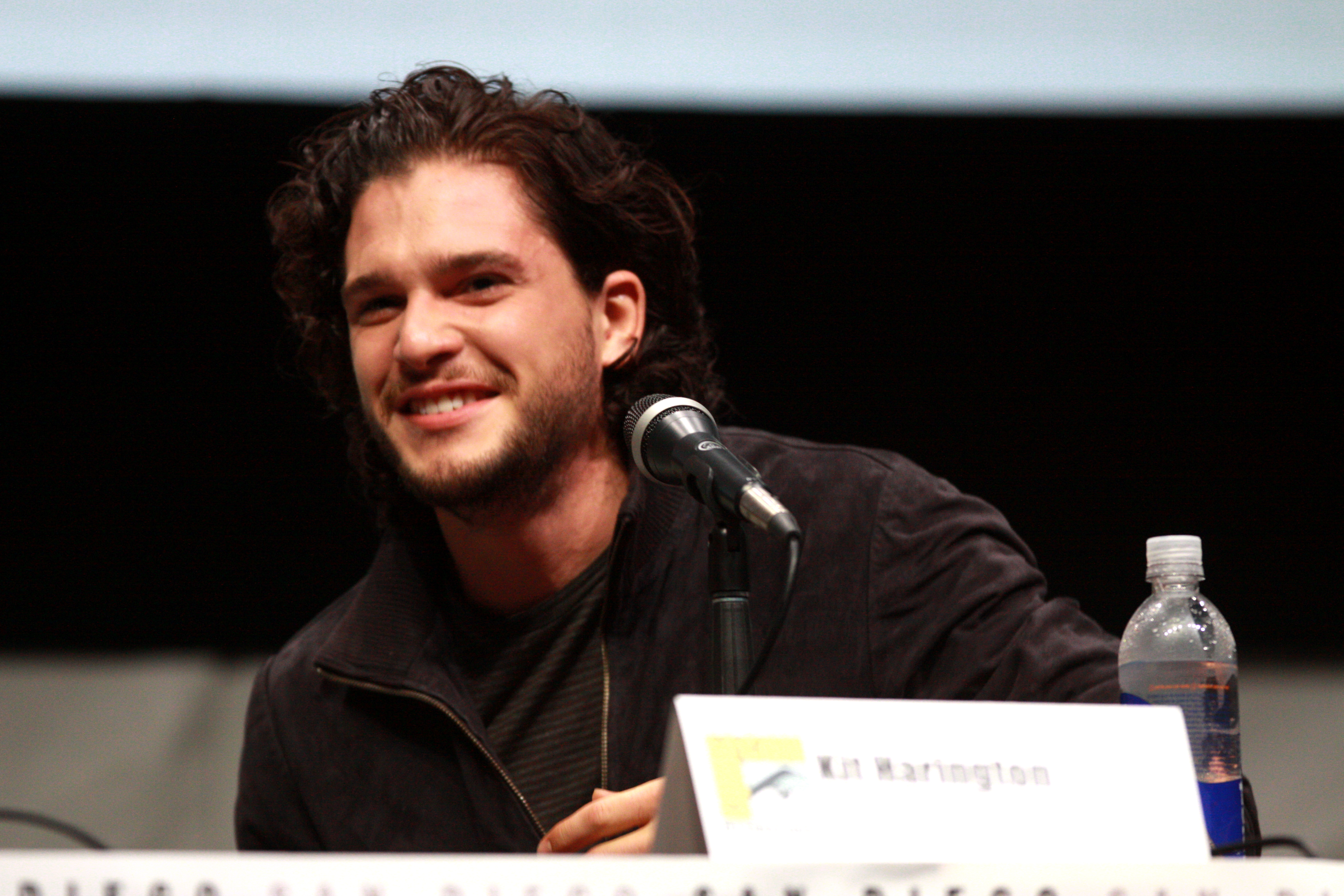The photo captures Kit Harington seated at a table with a name tag in front of him, reading "Kit Harington," although it's slightly out of focus. He is smiling widely and looks directly at the camera. In front of him, there's a bottle of water and a microphone. Kit is wearing a dark, zip-up jacket over a dark gray and black striped t-shirt. His hair, which is dark and somewhat wavy, falls to his shoulders and is slicked back. He also sports a short beard and mustache. The background of the image is predominantly black, with a gray-blue hue at the top and a grayish tone towards the bottom, suggesting the possible presence of a floor and curtains, although they are blurry and indistinct.